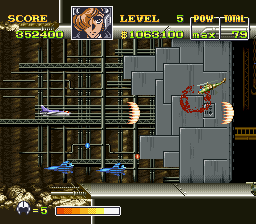This screenshot from a video game shows a bustling and intricate scene. At the top, a status bar displays the score of 352,400 and the player is currently on level 5. Additionally, there's a display of in-game currency amounting to $1,063,100, with a power maximum of 79. Dominating the scene is a room featuring irregularly shaped, rectangular, and square gray walls adorned with numerous greenish-metal pipes. Within this room, various elements are in motion, including two blue airplanes flying towards the left and multiple aircraft—white, purple, and possibly green helicopters—navigating through a grid of pipes. Also present are two unidentified entities that might be bats, parachutes, or additional planes, all heading to the right. Amidst these, a conspicuous rough-painted “O” or zero marks the gray wall. Toward the bottom, a black bar marked with a number 5 indicates the remaining lives, flanked by a life indicator displaying bars in red, orange, yellow, and white hues, as well as a flame-like symbol anchoring the dynamic atmosphere of the game.